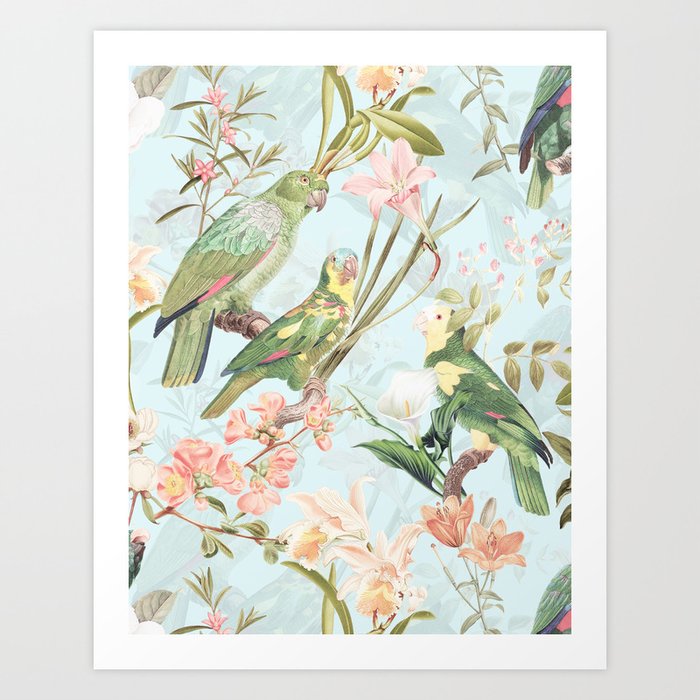The image displays a framed artwork, possibly a painting or a digital print, set against a light gray wall. The frame is plain white, accentuating the vintage, soft, and feminine colors of the piece. The background of the artwork itself is a very light eggshell blue, creating a serene backdrop for the vibrant yet subtly saturated elements. 

In the scene, three whole parrots prominently occupy the branches, with the edges of several other birds peeking in. The main central branch hosts two parrots: the upper one is predominantly green, with lighter green and blue-tinted wings, a white top area, and pink and black trim above the tail. The lower parrot on the same branch features a powder blue head, a pink beak, and a body that is mostly green with yellow feathers tipped in pink. On the adjacent branch, next to a calla lily, perches another parrot with a green body, yellow face, tan beak, and a touch of white above the beak.

Surrounding the parrots is an array of flowers in pink, peach, and yellow, adding to the rich, soft palette of the artwork. This detailed portrayal captures the delicate interaction between the vibrant birds and the abundant flora, showcasing a harmonious blend of nature’s beauty.